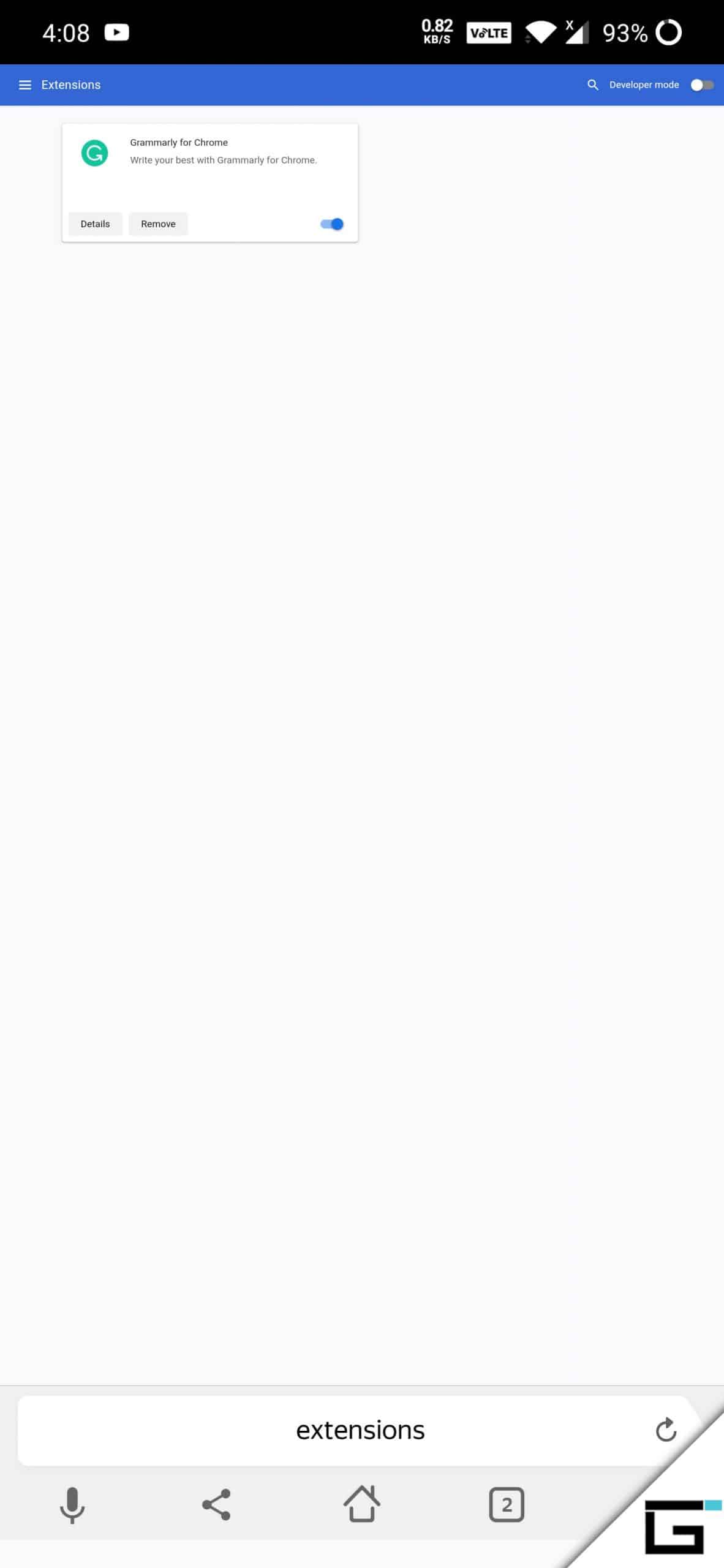A screenshot of a smartphone's screen displays various interface elements. At the top left, the time reads "4:08," and the right side shows a small notification icon linked to YouTube, indicating 0.82 KB of data. The Wi-Fi indicator shows no connection as denoted by a small 'X' above it, and the battery life is at 93%.

The phone appears to be in developer mode, and on a white screen, the display showcases a section titled "Grammarly for Chrome," with a message prompting the user to "Write your best with Grammarly for Chrome." Below this message are two buttons labeled "Details" and "Remove," both in gray with black font. A blue toggle button next to Grammarly indicates it is active. Grammarly's logo, a green circle with a white 'G' in the center, is also visible. At the bottom of the screen, the interface features buttons labeled "Extensions" and "Refresh," along with a white search bar.

Additional icons are present at the very bottom, including a microphone, share option, home button, a square with a number '2' inside, and another icon featuring a black 'G' isolated in the bottom right corner, sectioned off slightly from the others. The overall color scheme includes black, white, gray, blue, and green, but the predominant background color is white.